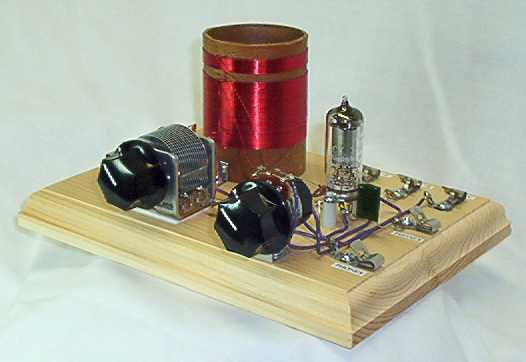The image appears to depict an old-fashioned memory board, potentially from a vintage electronic machine, mounted on a thick wooden base. The board is detailed with various gadgets and intricately connected components. Notably, there is a prominent cylinder with red coils on the upper backside, and the setup includes two black knobs on the front. Numerous silver pieces are present, along with light purple cords running through the assembly. The image also features a light bulb, wire connectors, and charging stations, all suggesting an electrical experiment or circuitry related to lighting. The board is placed on a white sheet, possibly for the purpose of photographing it for listing or documentation. Overall, this complex assembly of black and silver baubles, wires, and levers underscores its vintage and experimental nature.